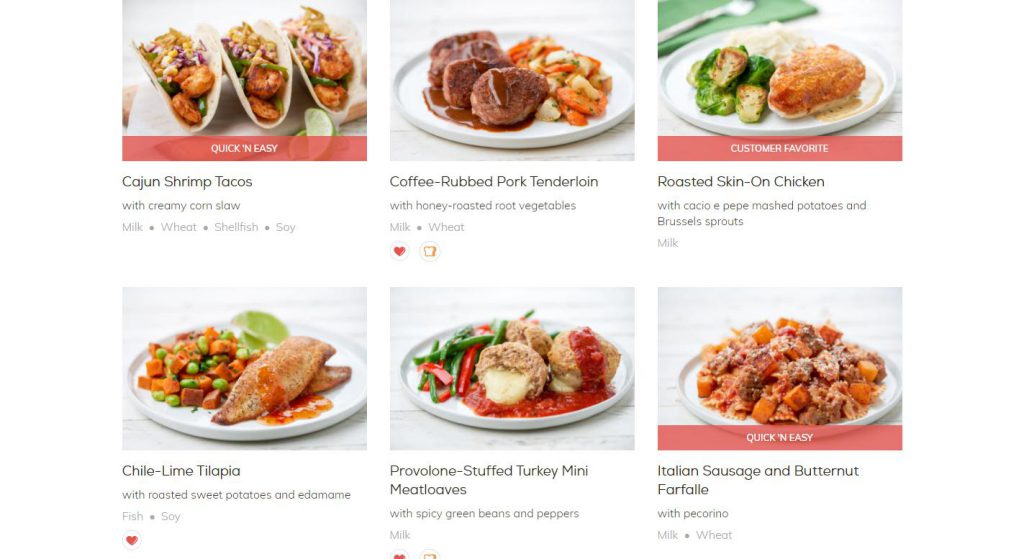The image depicts a vibrant and professionally designed website dedicated to recipes, featuring six distinct dishes. The recipes showcased are:

1. Cajun Shrimp Tacos
2. Coffee Rubbed Pork Tenderloin
3. Mustard Skin-on Chicken
4. Chili Lime Tilapia
5. Provolone Stuffed Turkey Mini Meat Loaves
6. Italian Sausage and Butternut Squash Fava

Three of these recipes are prominently highlighted with a red banner: two are labeled "Quick and Easy," while one is marked as a "Customer Favourite." 

This website appears to be from a meal kit service, providing not only the recipes but also all necessary ingredients and a detailed instruction card for each meal. The high-quality, professionally taken images display the dishes in a very appealing manner, each plated on plain white plates that are filled to the brim with vibrant and tasty-looking food. Each dish is accompanied by a concise description, enhancing the user’s experience by offering a glimpse of what to expect from the meal.

The visual presentation showcases a wide variety of meats and fishes, ensuring there is something to appeal to diverse culinary preferences.